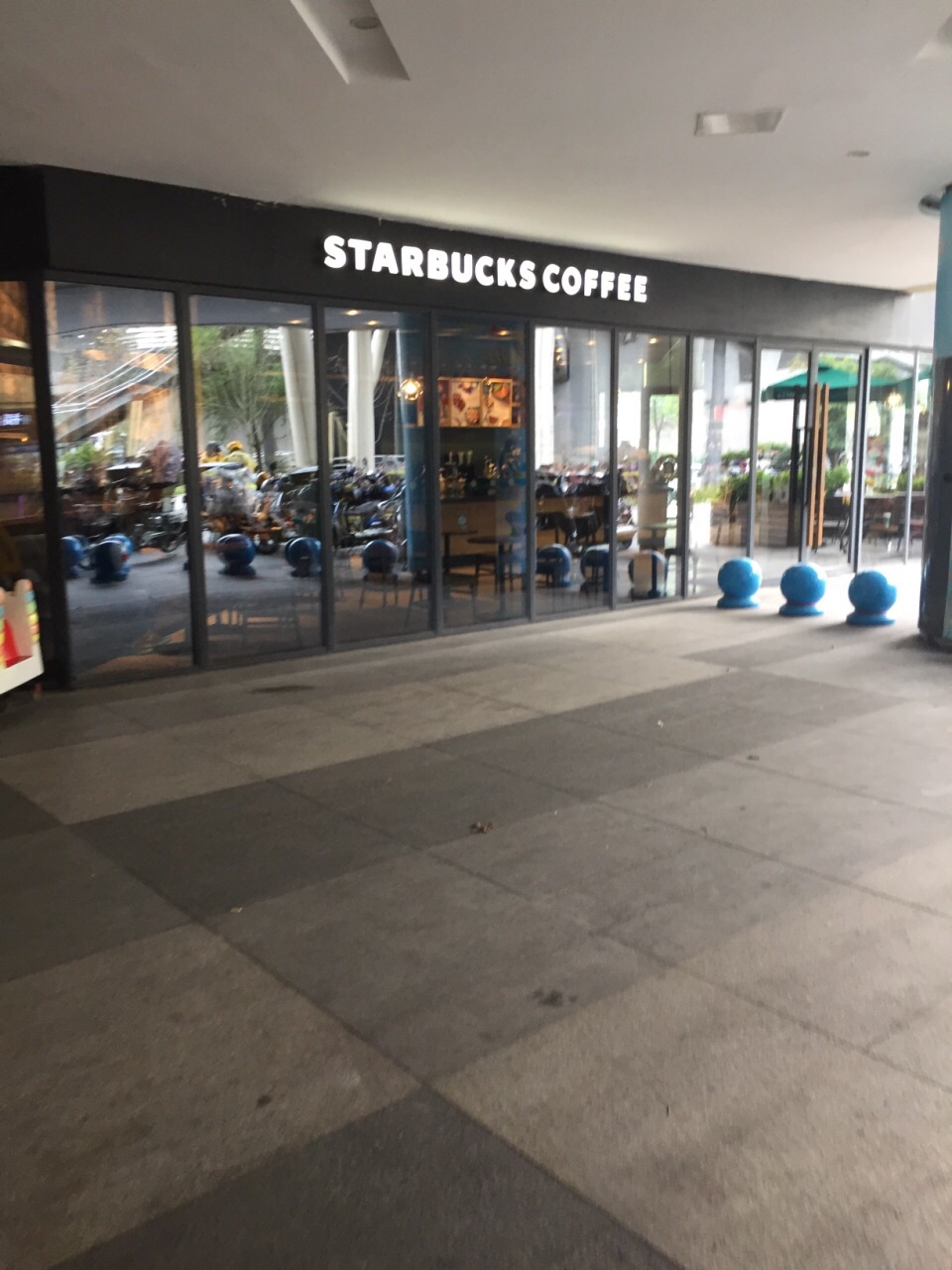This image captures the exterior of a Starbucks Coffee shop, viewed from underneath its veranda. The sign "Starbucks Coffee" is prominently displayed in crisp white letters against a black background over the front entrance. Below the sign, large black-framed windows make up much of the facade, allowing a peek into the dimly-lit interior where more chairs are arranged. Under the white ceiling of the veranda, several lights provide illumination. To the right, three blue poles stand on the grey tiled ground, which has a mix of light and dark grey squares. A single dry brown leaf lies on the ground in the center of the image. Further to the right, beyond the blue poles, there are outdoor brown chairs arranged in front of the building. The pillars separating the glass panels of the Starbucks are also black. Reflections in the window include the blue poles and a hint of a blue-tinted image, adding to the scene's complexity.